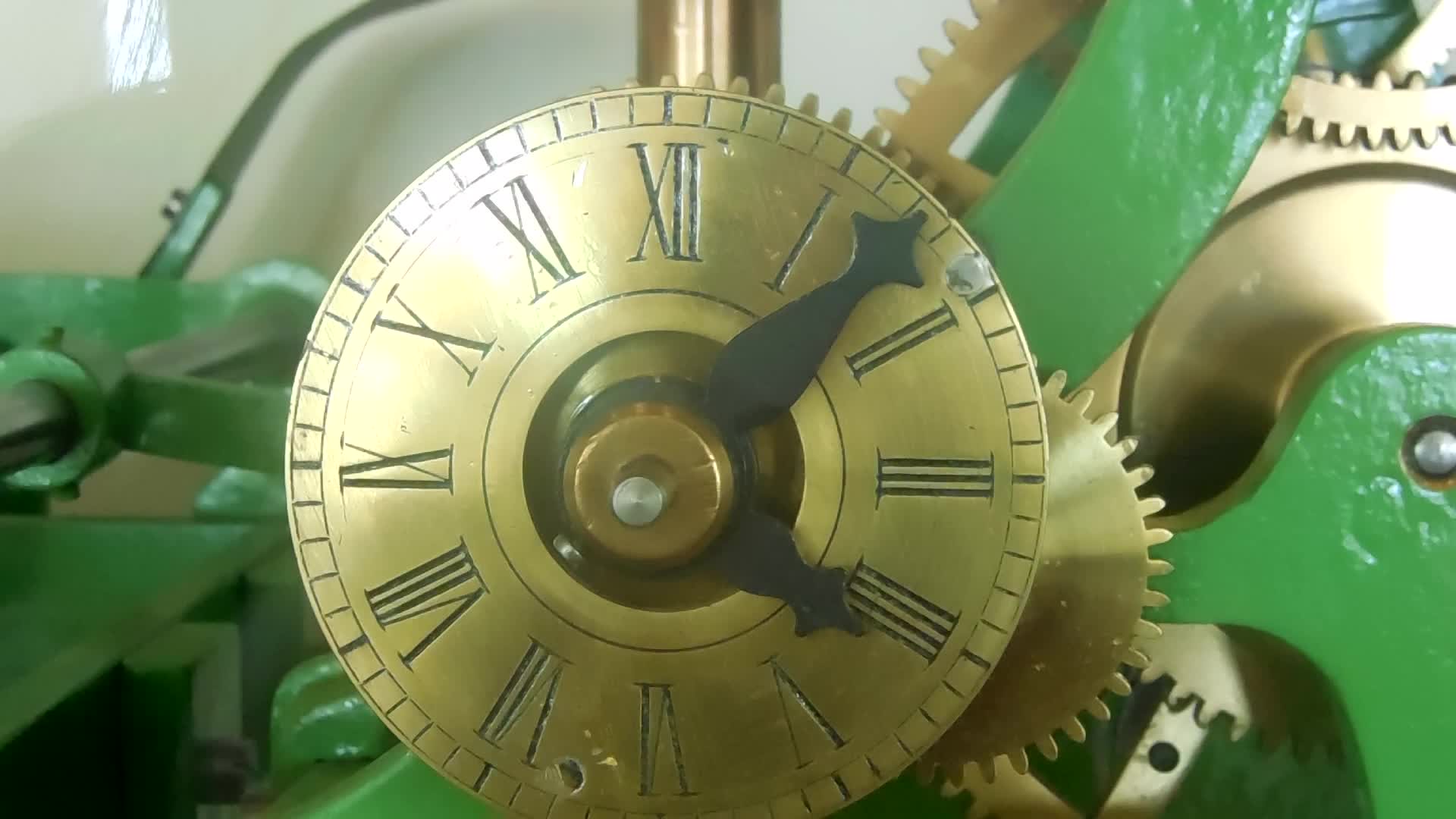The photograph captures a detailed view of a clock's face, which is prominently centered within the frame. The clock features Roman numerals marking each hour, while the minute markers are detailed points around the edge of the clock face. Surrounding the clock face are various screws and metal components, offering a glimpse into the intricate inner workings of the timepiece. The predominant colors in the image include shades of green, a bronzy metal hue, and white, contributing to an overall antique and mechanical aesthetic. The setting appears to be in a building, potentially a museum or train station, suggested by the subtle reflections visible in the background, possibly from a window or glass casing. The clock's intricate design and aged materials evoke a sense of history and craftsmanship.